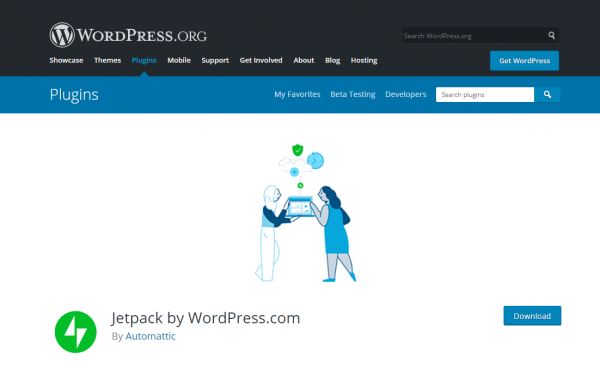The webpage displayed is from WordPress.org, featuring a navigation bar that stretches across the top of the screen. This navigation bar is distinguished by its gray background with white text. Located at the far left of the bar, the WordPress.org logo is prominently displayed. Adjacent to the logo, small menu items appear, reading left to right: Showcase, Themes, Plugins, Mobile, Support, Get Involved, About, Blog, and Hosting. The "Plugins" menu is notably highlighted in blue, with a dropdown arrow next to it. Below this highlighted menu, a secondary blue bar also labeled "Plugins" extends horizontally. Toward the middle-right portion of this bar, additional options are listed: My Favorites, Beta Testing, Developers, along with a search box for user convenience.

Dominating the main section of the screen is an illustrative image that appears hand-drawn in a simple, stock style. The illustration features a woman and a man standing side by side, each holding one side of a laptop computer. Emanating from the top of the laptop are multiple bubbles, with recognizable icons inside. One bubble contains a clock, another shows a green shield with a check mark, though the remaining icons are indistinct.

Below this central image, at the bottom left corner of the main content area, there is a green circle encompassing two white triangles pointing in opposite directions—one upward and one downward. Next to this icon, the text reads "Jetpack by WordPress.com by Automattic." On the far right side of the screen, a blue button is prominently labeled "Download."